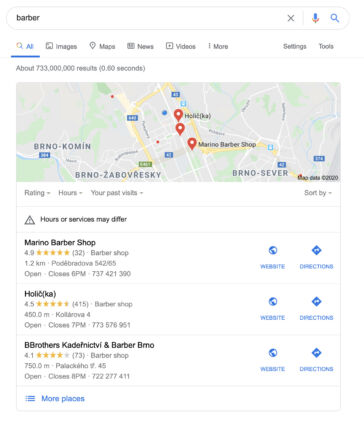This is a detailed caption of a Google search results page screenshot. The search query "barber" is entered in black text within the white search bar at the top. The interface displays various navigation options below, including "All," "Images," "Maps," "News," "Videos," "More," "Settings," and "Tools." The "All" tab is selected, indicated by blue underlining. In gray text, the search results total "About 733 million results (0.60 seconds)."

Below, there is a map showing a central or eastern European town with three red pins. The map includes a label for "Merino Barbershop" on one of the pins and the note "Map data ©2020" in the bottom right corner. Beneath the map, options for filtering the results such as "Rating," "Hours," "Your past visits," and "Sort by" are available. There's also a warning symbol featuring a black triangle with an exclamation point inside, stating "Hours of services may differ."

The list of three barbershops follows:
1. "Merino Barbershop" is rated 4.9 stars, located 1.2 kilometers away, closing at 6 p.m.; contact number 737-421-390.
2. "Holishka" is rated 4.5 stars, located 450 meters away, closing at 7 p.m.; contact number 773-578-951.
3. "B Brothers Katerinic TV and Barbara Verno" is rated 4.1 stars, located 750 meters away, closing at 8 p.m.; contact number 722-277-411.